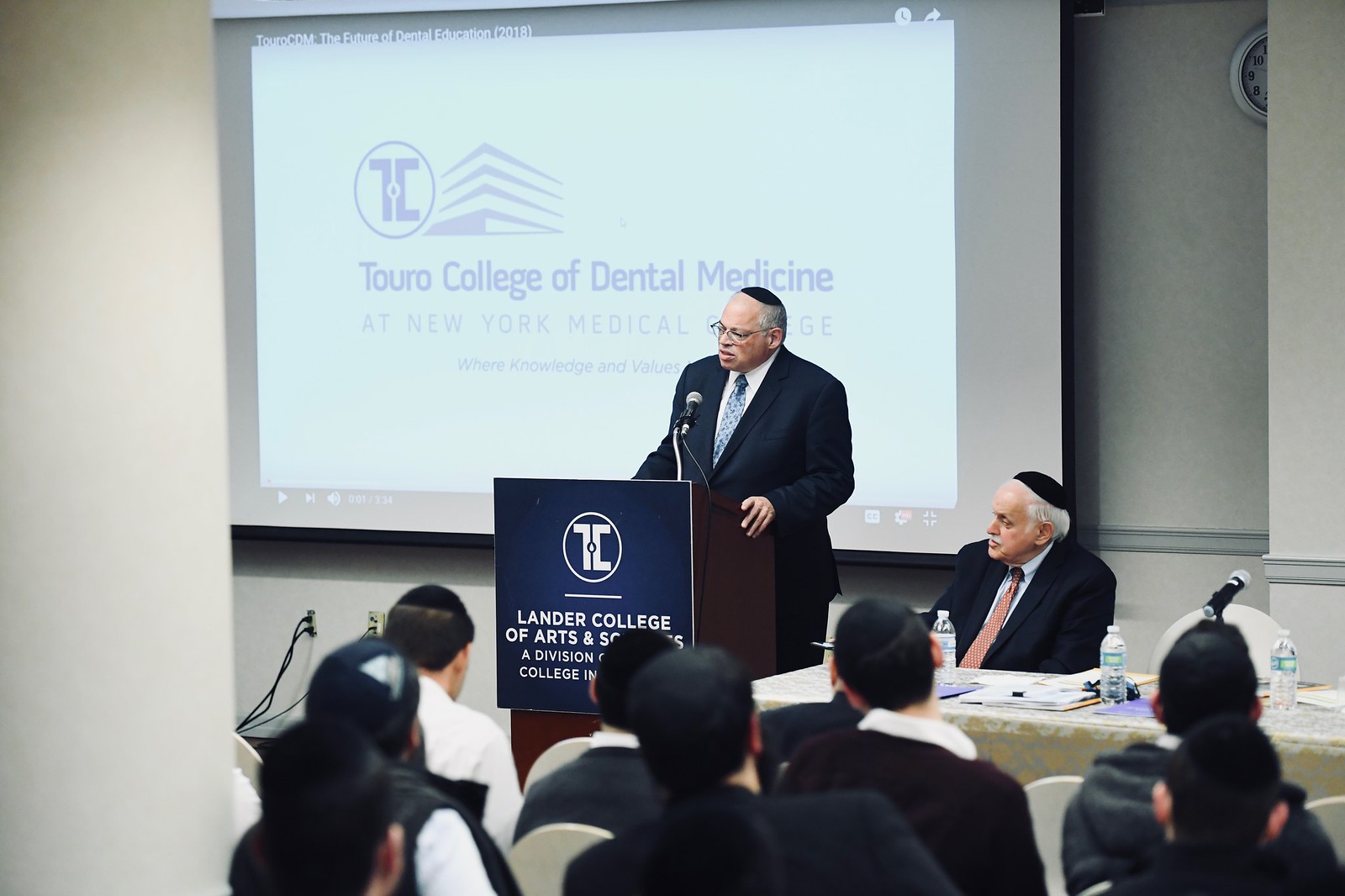In the image, a man stands at a dark brown podium delivering a lecture, likely at a college. Behind him, a screen projects text that reads "Touro College of Dental Medicine at New York Medical College." The podium features a blue sign that partially reads "Lander College of Arts and Science." The speaker, dressed in a black suit, white collared shirt, and blue patterned tie, also dons glasses and a black yarmulke. He speaks into a microphone positioned on the podium. Adjacent to him, another man in a black suit with a red patterned tie and a black yarmulke sits at a table covered with a light tablecloth, which holds water bottles and additional microphones. The audience, seen from behind, includes several men wearing dark suits, white shirts, and yarmulkes, suggesting the event is at a Jewish institution. The room is simply decorated with gray and white walls, creating a formal and focused atmosphere for the lecture.